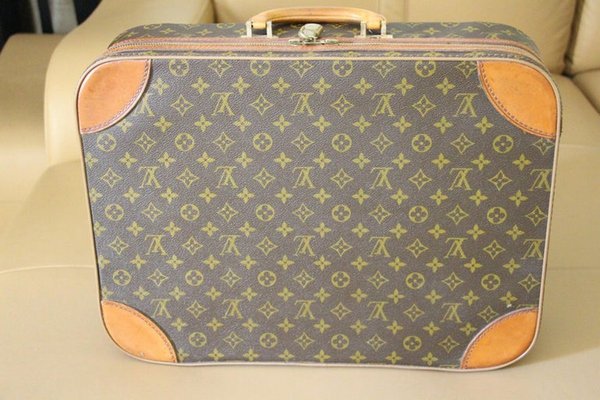This image features a vintage Louis Vuitton suitcase prominently displayed in the foreground. The suitcase, which lacks wheels and is crafted to be carried by a handle, is medium-sized and exhibits signs of age, giving it an antique appearance. Its design showcases the iconic Louis Vuitton logo interspersed with star shapes, round shapes, crosses, and fleur-de-lis, all set against a black background. Each corner of the suitcase is reinforced with semi-circular brown leather patches, matching the brown wooden handle positioned at the top near the visible zipper. The suitcase is placed on what appears to be a cream-colored leather couch, but the couch isn't fully visible due to the close-up focus on the suitcase. The setting suggests an intimate, possibly staged arrangement, hinting that the photo might have been taken to showcase the luggage for sale.